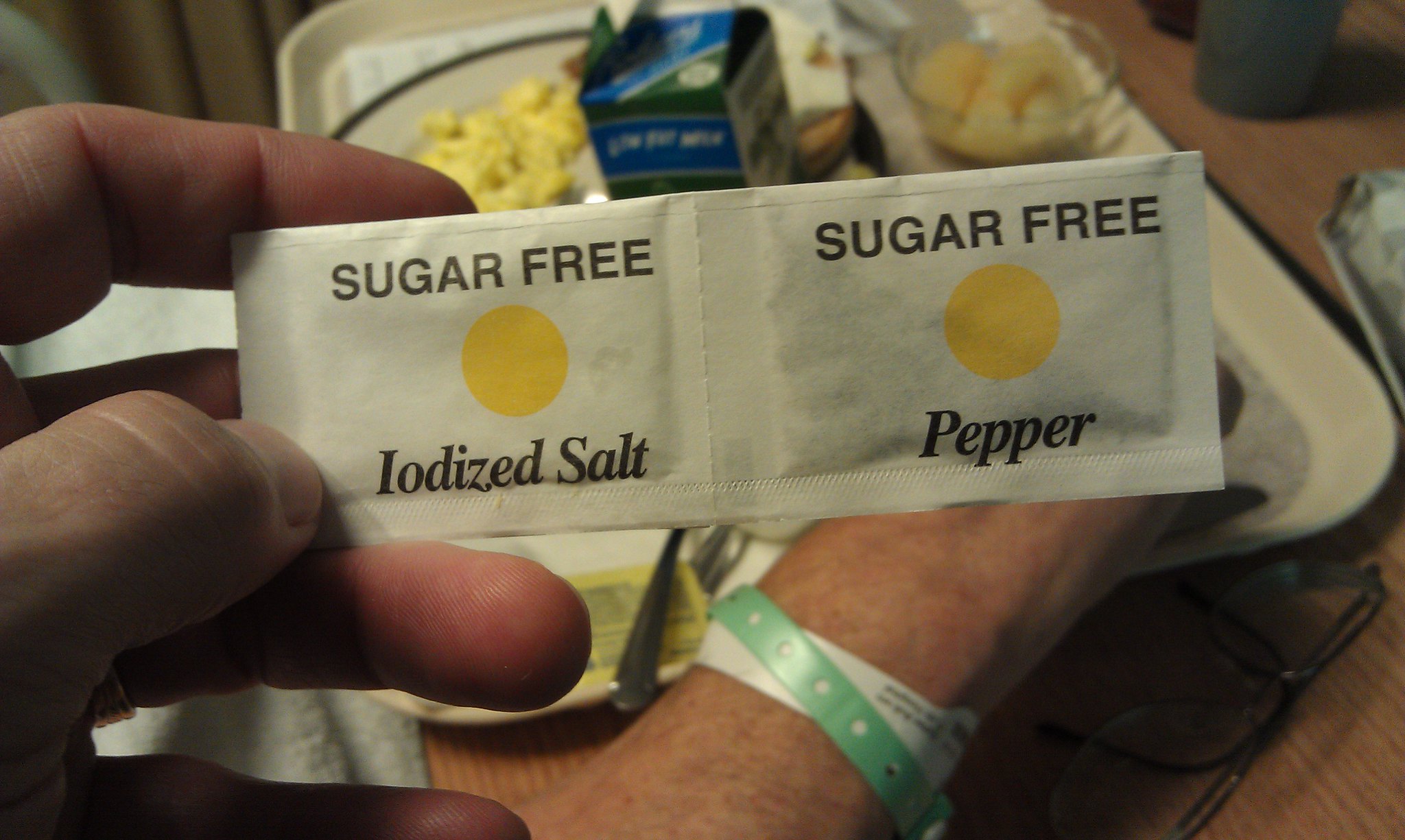In this photo, likely taken at a festival or potentially at a hospital, the focus is on a close-up of a table laid out with a meal. A tray holds a dinner plate with an assortment of food items, accompanied by a small glass bowl filled with fruit. Intriguingly, part of the scene includes a person's partially visible hands; their right hand is hidden behind several sachets, held by the left.

The sachets, connected together and held in the left hand, catch the eye. They are both white with a distinctive yellow dot in the middle. Labels on the sachets read "sugar-free iodised salt" and "sugar-free pepper." The person appears to be examining these packets closely. A festival or hospital wristband is noticeable on the individual's wrist, suggesting the setting could be either a lively event or a medical environment, hinting that the sugar-free seasoning might be a dietary requirement. The angle of the photograph provides a personal, first-person perspective of the scene.